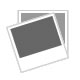This highly detailed photograph depicts two extremely rusty bolts positioned side by side on a scratched and worn metal surface. The aged surface has numerous divots and scratches, indicating significant wear, and appears brighter at the bottom due to the light source emanating from below. The bolts, angled from the top left to the bottom right of the image, are several inches long with hexagonal heads and large washers at the top, though these elements are partially obscured as they face away from the viewer. The bolts are completely encrusted with rust, and their threads extend approximately two-thirds of the way up, leaving the upper third and the bottom few millimeters smooth and unthreaded. The extensive rust and oxidation suggest they are old and no longer functional, lying alone without any markings or hands holding them. The close-up nature of the photograph makes the bolts appear larger than their actual size, amplifying their worn and aged condition.